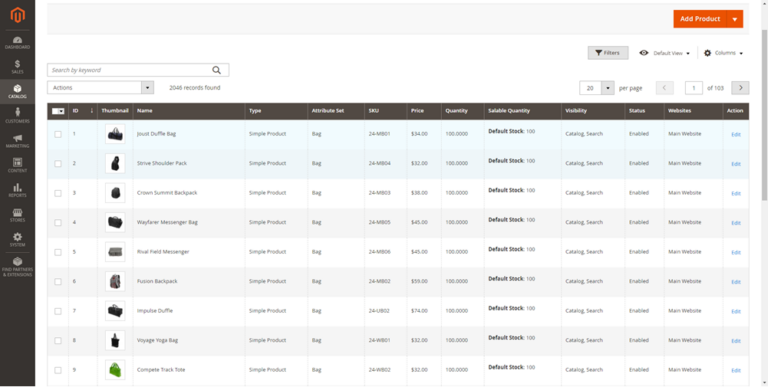The image is a screenshot of a stock management page on a website, likely from the backend view. The screenshot encompasses a large portion of the page, making specific details somewhat difficult to discern. The page displays a catalog of various bags including duffel bags, shoulder packs, backpacks, messenger bags, a tote or yoga bag, and a track bag. Most of these bags appear to be black, with one green track bag, and a messenger bag and a backpack in a grayish color.

Pricing information is visible, although not entirely clear due to the zoom level of the screenshot. Prices seem to range between approximately $30 and $75. The quantity for each item listed appears to be set at 100,000 units.

Additional features on this page include search filters, options to add more products, and a sidebar on the left with multiple categories available for selection beyond the catalog view.